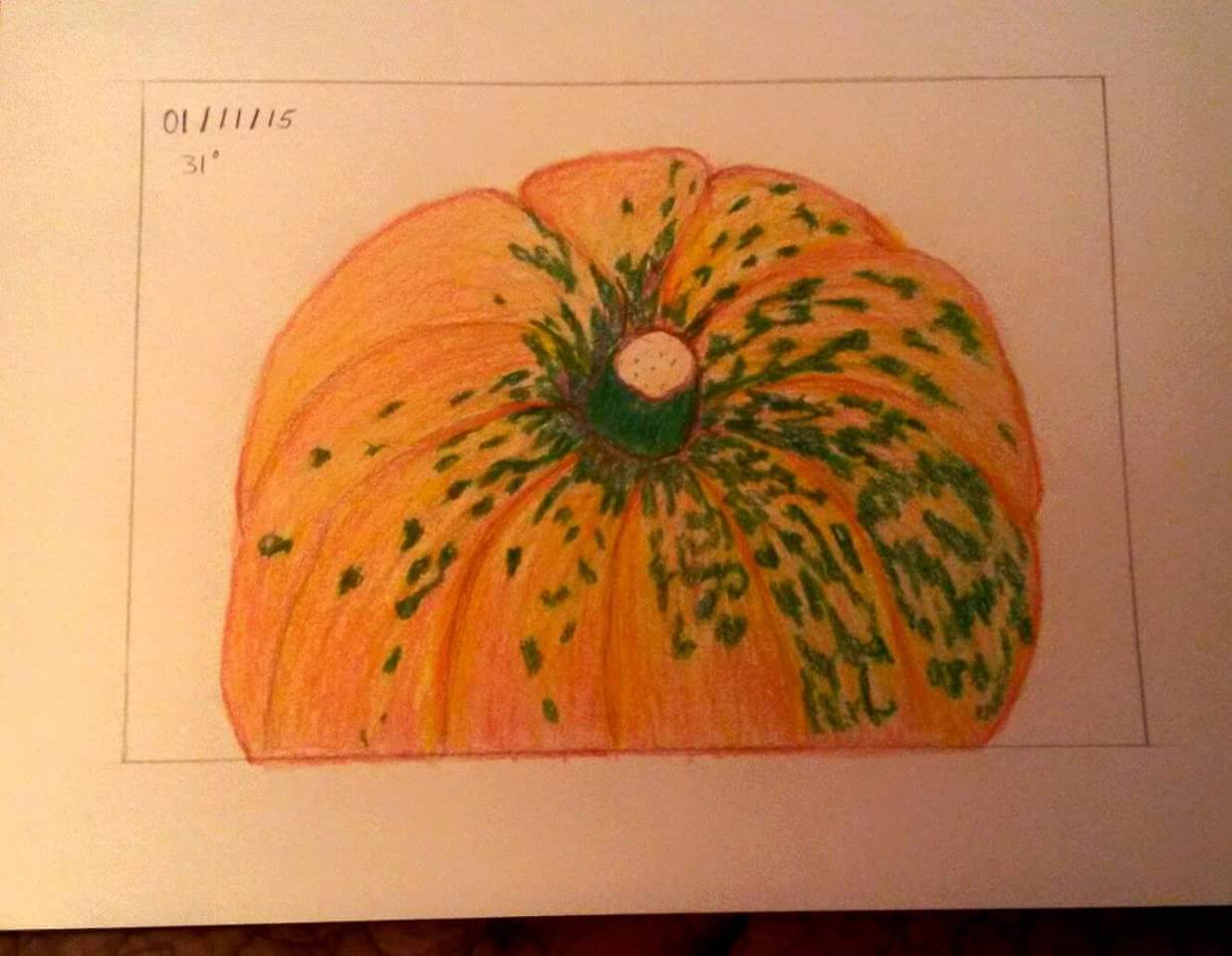The image depicts a detailed hand-drawn pumpkin filling most of the page, rendered in what appears to be a middle school student's style using colored pencils. The pumpkin is primarily orange with green spots scattered across its skin, indicating areas that are still ripening. The green stalk, located at the top center, is depicted with a creamy white center visible where it has been cut. The pumpkin is segmented with grooves characteristic of its outer shell. The perspective is from a slightly angled top-down view. The drawing is framed within a hand-drawn pencil rectangle on white or cream-colored paper, seen against a darker surface, possibly a tabletop. The overall colors in the photograph appear slightly dull due to the yellowish lighting. In the upper left-hand corner of the rectangle, the numbers "01 11 11 15" are written, followed by "31°" below them.